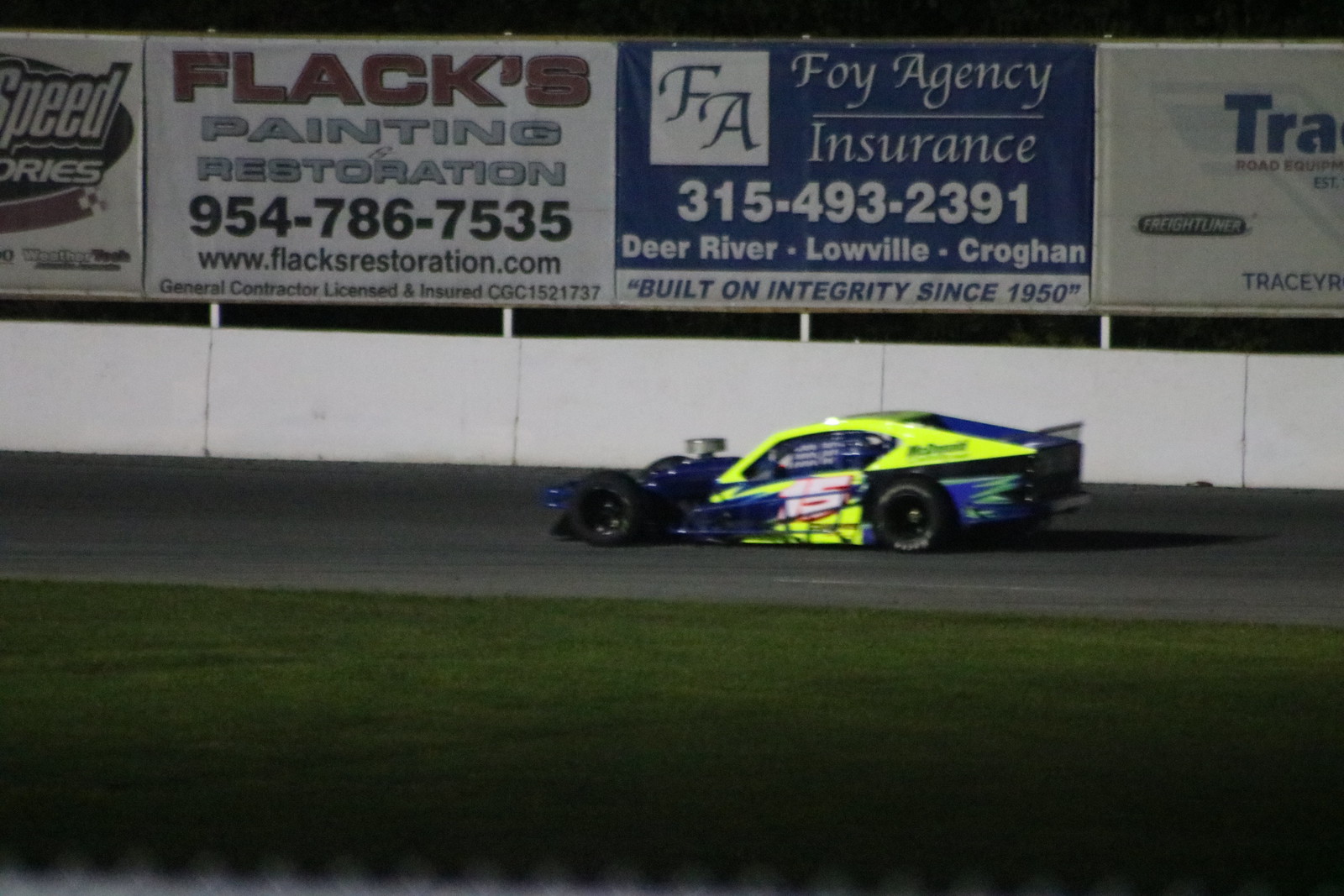In this detailed image, a vibrant race car is speeding from right to left on a racetrack. The car, predominantly blue with neon green and yellow accents, features a white number 15 on its door and green flames near the back. Notably, the vehicle appears to have some netting on the door and an exposed motor at the front, indicating a high-performance, perhaps custom-built race car. 

The bottom portion of the image shows a grassy infield and the dark black asphalt track, bordered by a white cement sidewall. Above this wall runs a series of advertisements. From left to right, the topmost ad partially visible says "Speed" within a circular design. Adjacent to this is a more prominent white background ad with red text reading "Flax." Below it, in gray text, are the words "Painting Restoration." The ad continues with a black phone number "954-786-7535," followed by the website "www.flaxrestoration.com," and proclaims "General Contractor Licensed and Insured CGC 1521737."

To the right, another prominent blue-background ad displays in white letters "Foy Agency Insurance" along with its contact details. Lastly, to the far right, albeit a bit faded and unclear, there are additional, less legible advertisements. The scene vividly captures the dynamic action of the race car contrasted against the commercial backdrop of the racetrack's advertising.